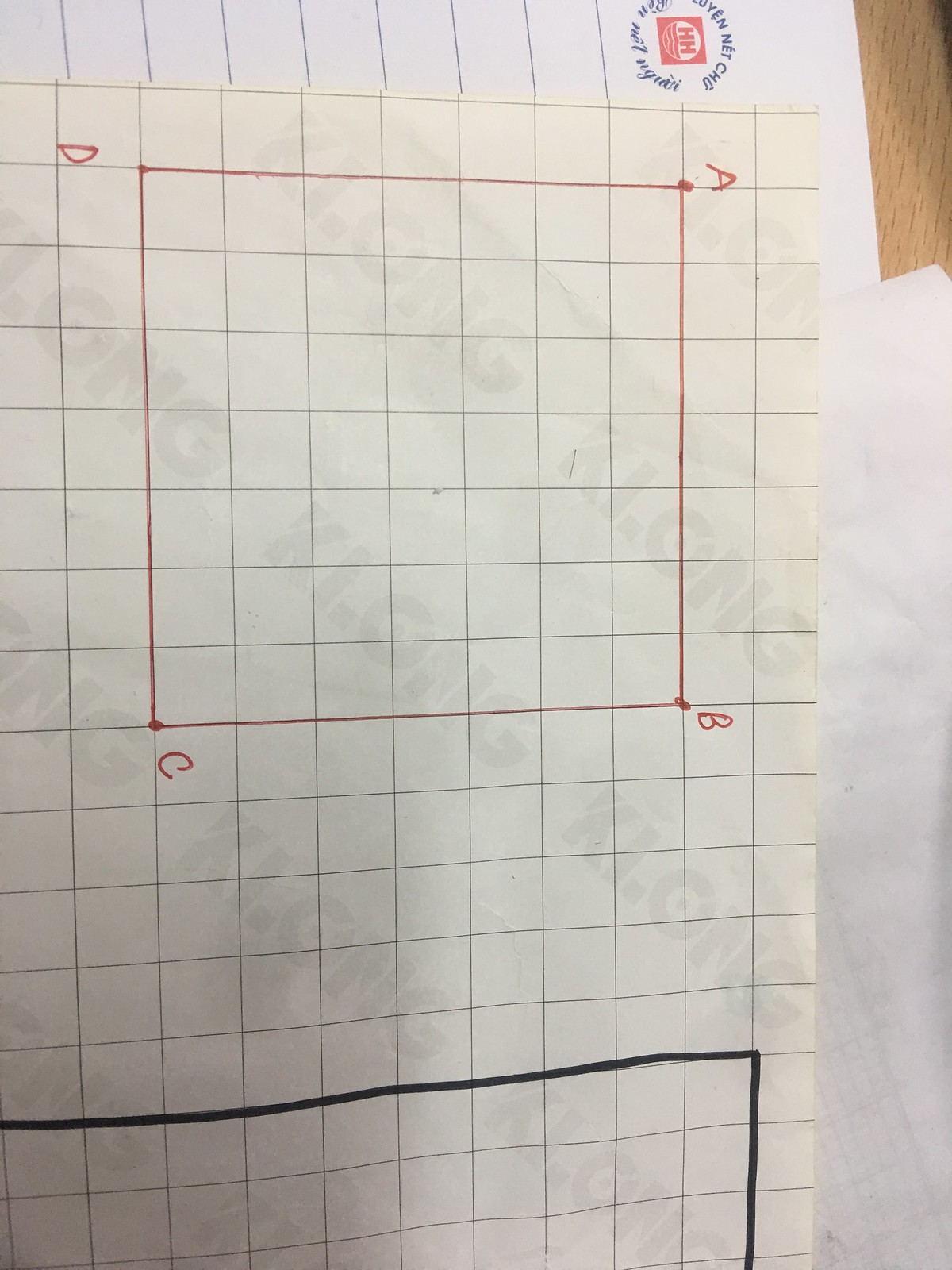The image depicts a piece of yellowish graph paper with a one-centimeter grid marked by black lines. The paper is oriented sideways at a 90-degree angle. Near the top, there is a square formed by four red felt pen lines, with dots at each corner labeled "A," "B," "C," and "D" in red ink. 

Approximately five grids down from the top, a thick black line extends horizontally across the paper from the left edge, nearly reaching the right side, before descending vertically for three grids.

Adjacent to the top, there is a smaller white sheet of paper displaying the symbol "HH" in red, surrounded by a blue circle with indiscernible text, possibly in Chinese or Vietnamese, which is not entirely legible. Another piece of white paper is visible behind the graph paper.

A faint watermark that reads "K-L-O-N-G" is discernible on the graph paper, adding an additional layer of detail to the image.